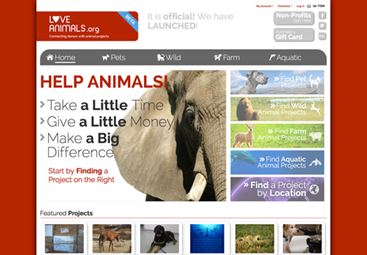The image showcases a very compact website interface with a red vertical border on the left and right sides. In the top-left corner, the website's header "loveanimals.org" is displayed in white text on a red background. Just to the right, a gray text message reads "It's official. We have launched," accompanied by two small gray rectangles, which may represent buttons or icons, and tiny black text categories in the top-right corner.

Directly below, there are five main navigation tabs labeled "Home," "Pets," "Wild," "Farm," and "Aquatic," all in white text on a gray background. Underneath this navigation menu, a prominent red text caption reads "Help Animals." Further down, a motivational message in black text urges viewers to "take a little time, give a little money, and make a big difference," followed by a call to action stating "Start by finding a project."

The main content area of the website features a section with five project options, each represented by a background of varying colors: the top option in gray and blue, the second in tan and green, the third in green, the fourth in blue, and the fifth in purple. At the very bottom, the section titled "Featured Projects" is highlighted by six square images, though their specific details are not visible. The central part of the webpage maintains a predominantly white background, framing all the elements within this detailed website layout.